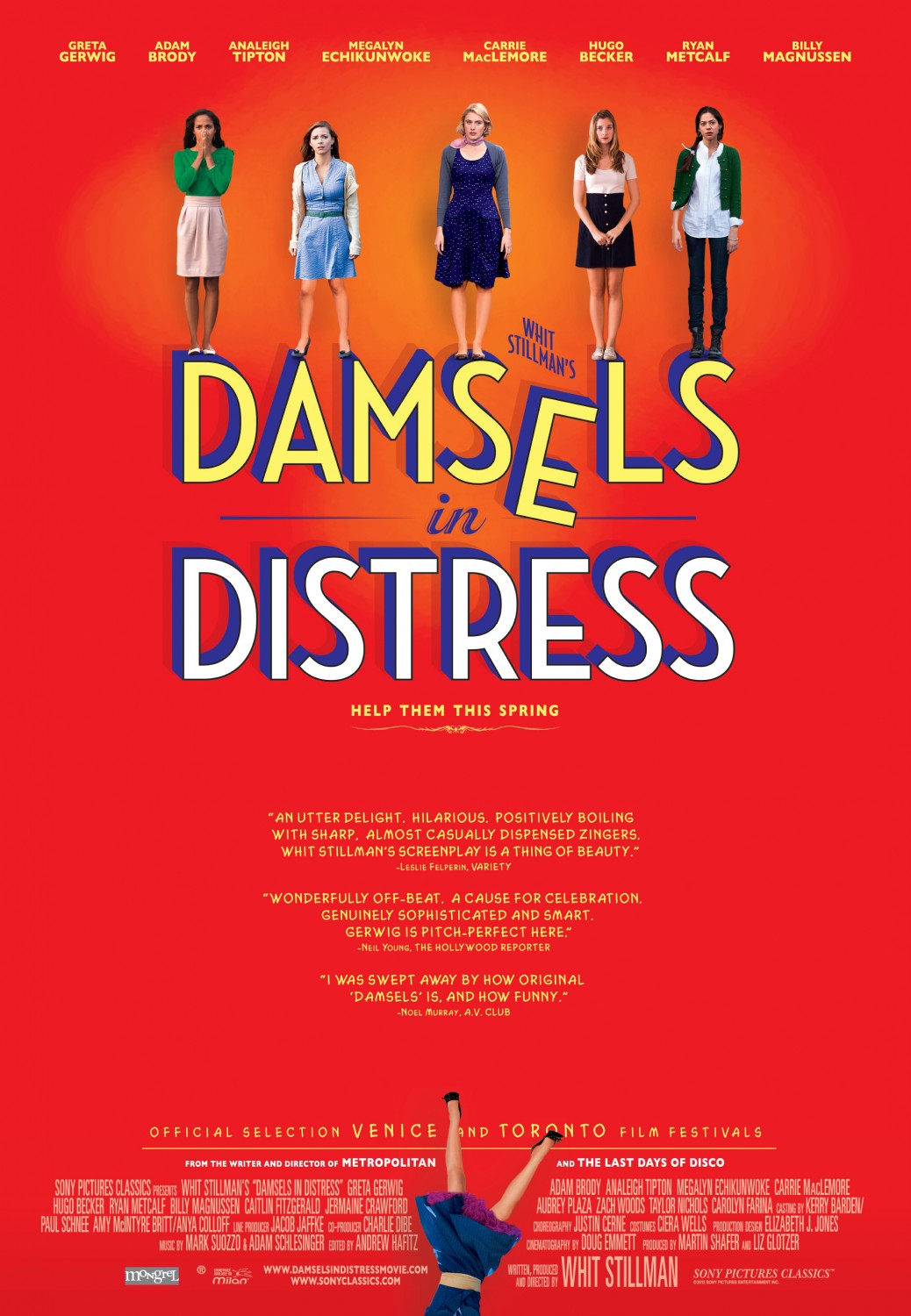The movie poster for "Damsels in Distress" by Whit Stillman features a light orange background transitioning to a darker red-orange towards the edges. The title "Damsels in Distress" is prominently displayed in large, 3D, blue-highlighted letters at the center. Standing atop these letters are the five main actresses, facing the camera in various outfits. 

From left to right: a young black woman with long hair, wearing a green top and white pencil skirt; a young woman with long brown hair in a one-piece blue dress; a taller blonde woman in a dark blue dress with a shawl; another young woman resembling a waitress in a white top and dark blue skirt; and an androgynous woman with a green jacket over a white shirt and pants.

Above the actresses, the names of the cast members are listed: Greta Gerwig, Adam Brody, Analeigh Tipton, Megalyn Echikunwoke, Carrie MacLemore, Ryan Metcalf, Billy Magnussen, and Hugo Becker. At the bottom, the tagline reads "Help Them This Spring," followed by blurbs in light yellow font and the note "Official Selection: Venice and Toronto Film Festivals." Additionally, a depiction of a woman stands upside-down with her legs and blue skirt partially cropped out of the image, emphasizing the film's quirky and playful tone.